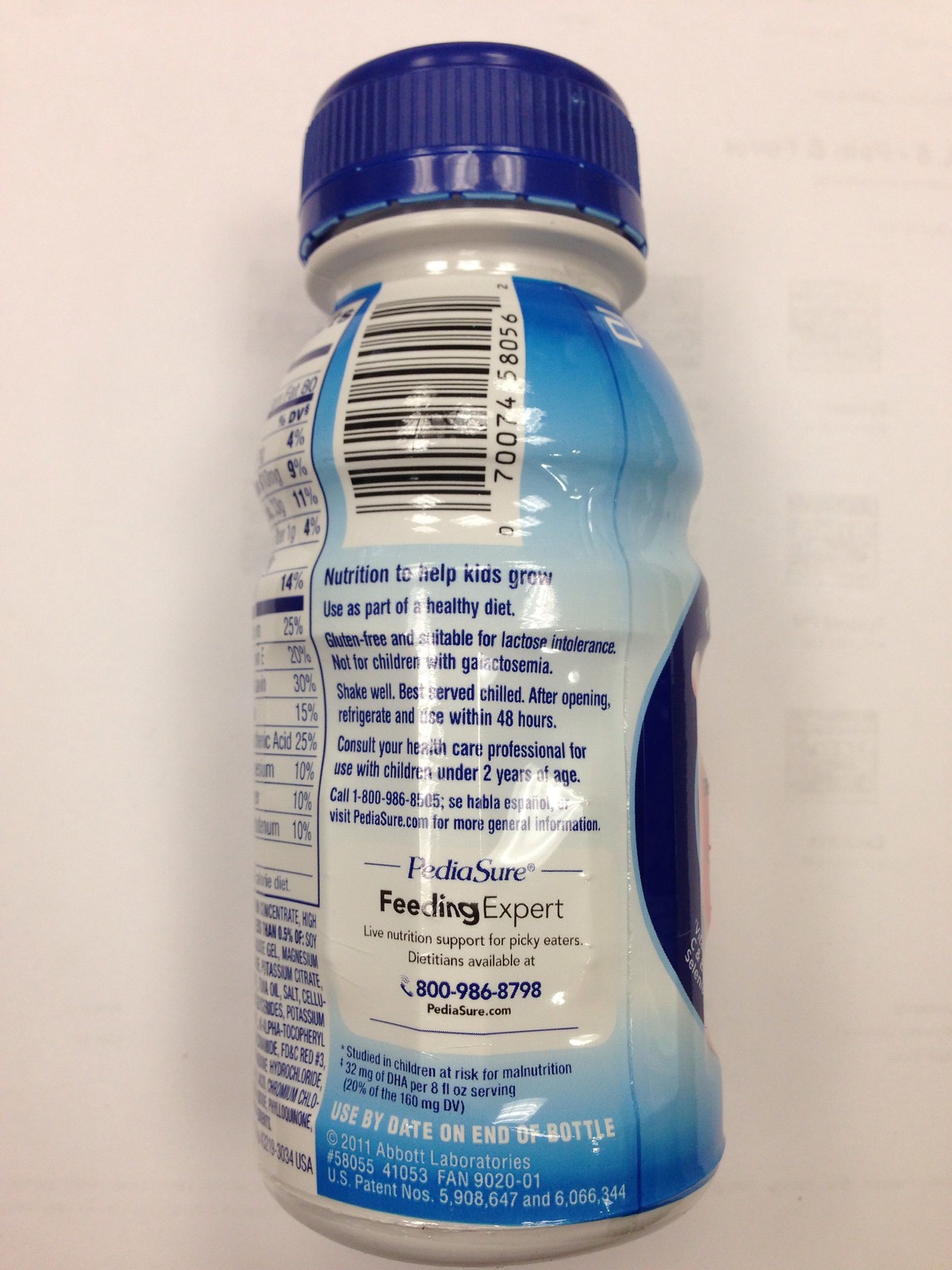This image depicts a close-up of a PediaSure bottle laying flat on a slightly pink-beige, off-white surface. The plastic bottle features a dark blue lid and a detailed, blue and white label. The upper portion of the label, which extends beyond the frame, includes a variety of information—some of which is partially obscured. Prominently displayed on the label is a white rectangle containing a black and white UPC barcode. 

Below the barcode, there is notable dark blue text set against a white and dark blue background, stating, "Nutrition to help kids grow," with light reflections across the text. Additional text advises that the product is gluten-free, suitable for lactose intolerance, but not for children with galactosemia. Instructions suggest shaking well, serving chilled, and refrigerating after opening, with usage recommended within 48 hours. A cautionary note emphasizes consulting a healthcare professional for use in children under two years old and provides a customer service number: 1-800-986-8505.

The label identifies PediaSure as the "Feeding Expert" and includes the same phone number again along with a use-by date specified at the label's end. In the visible portion of the label's back, nutrition information and ingredients are listed. In the background of the image, faint black markings resembling QR codes or scannable elements can be discerned through the paper's translucency.